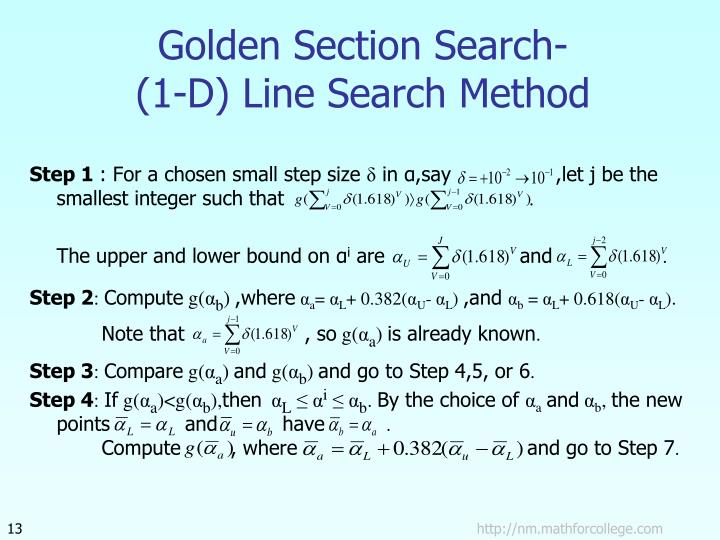The image is a detailed instructional slide with a light blue background, transitioning to a lighter shade towards the bottom. The centered, two-row title at the top is in blue text, reading "Golden Section Search - (1-D) Line Search Method." Below the title, four steps labeled in black text as Step 1 through Step 4, provide a comprehensive guide involving various numerical equations and mathematical figures. Step 1 begins with the phrase "for a chosen small step size," followed by additional detailed instructions. The bottom left corner shows the black number 13, signifying this is the 13th slide, while the bottom right corner features a grey watermark linking to the website http nm.mathforcollege.com.